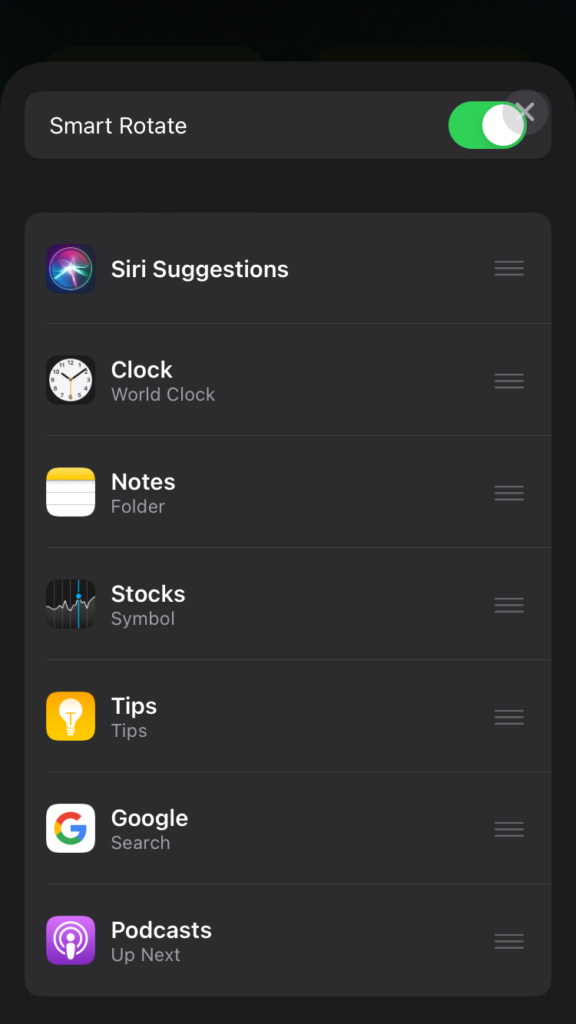This is a screenshot captured from a cell phone displaying a black background with white text. At the top, the text reads "Smart Rotate" accompanied by a slider button that is toggled on. Below this, there is a section titled "Siri Suggestions," featuring a circular icon of a glowing multicolored circle. 

The screen lists multiple icons and their respective labels:

1. **Clock (World Clock)**: Represented by an icon of a white clock with black hands.
2. **Notes Folder**: Indicated by an icon resembling a piece of paper.
3. **Stocks**: Denoted by a black icon displaying a white spiky graph.
4. **Tips**: Shown next to a yellow icon with a white light bulb in the center.
5. **Google Search**: Accompanied by the Google "G" logo, which consists of red, yellow, green, and blue segments.
6. **Podcasts (Up Next)**: Depicted by a purple icon featuring a microphone surrounded by two concentric circles.

The image is taller than it is wide and lacks any photographic elements, people, animals, birds, plants, flowers, trees, or airplanes.